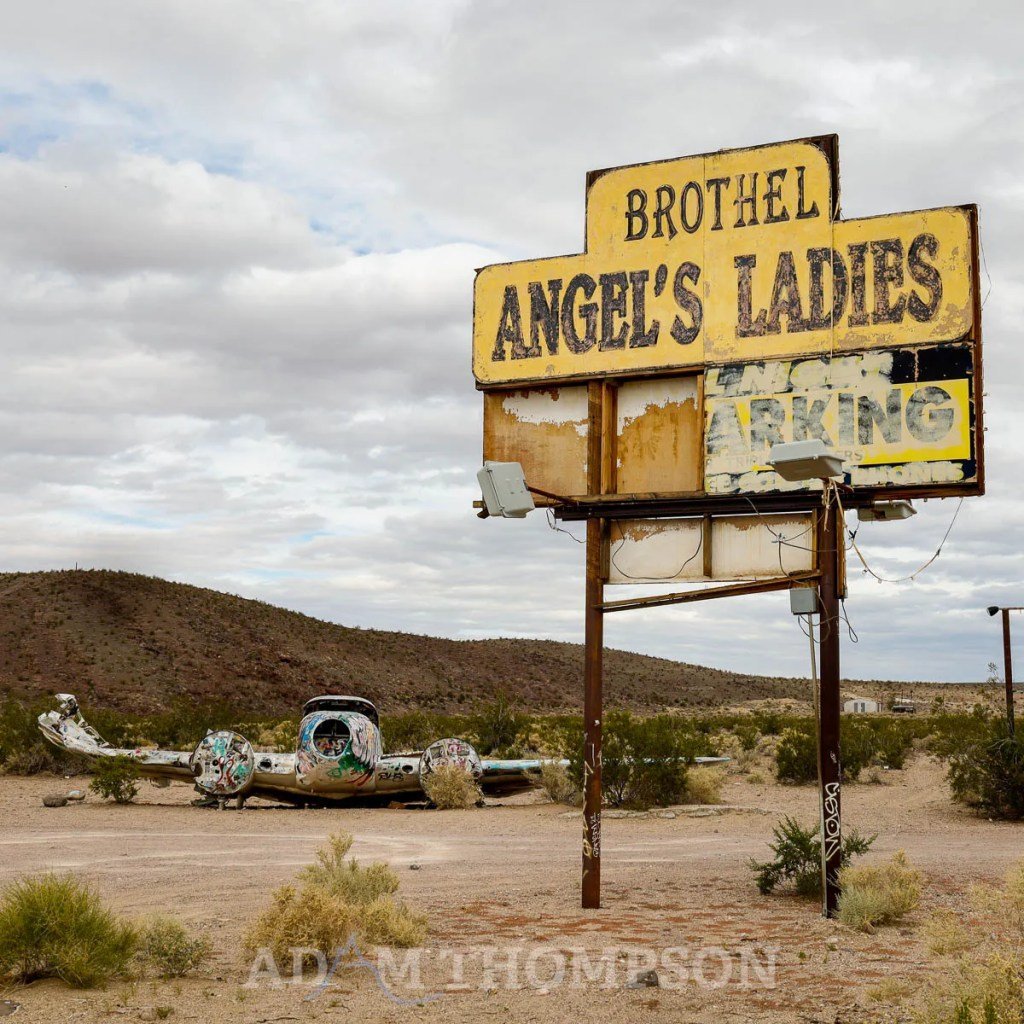In this evocative color photograph set in a deserted landscape, a dilapidated yellow and black billboard demands attention. The highly weathered sign reads "brothel, angels, ladies," with the bottom half torn away, and only fragments of the phrase "all night parking" remaining. Supported by wooden posts, this relic from a bygone era stands on a dirt surface adorned with sparse shrubs. Just behind the sign lies the wreckage of an abandoned, graffiti-covered airplane, stripped of its propellers, adding to the scene's desolate charm. Surrounding the sign, the expanse unfolds into a barren desert terrain dotted with greenery, while a distant brown hillside and a small white house occupy the horizon. Overhead, a mostly cloudy sky permits just slivers of blue to peek through, intensifying the sense of isolation. In the bottom right corner, a lone telephone pole stands as a silent witness to the past. At the very base of the image, the watermark "ADM Thompson" is subtly engraved, grounding this nostalgic snapshot of abandonment that evokes the feeling of an album cover or part of a photo series.